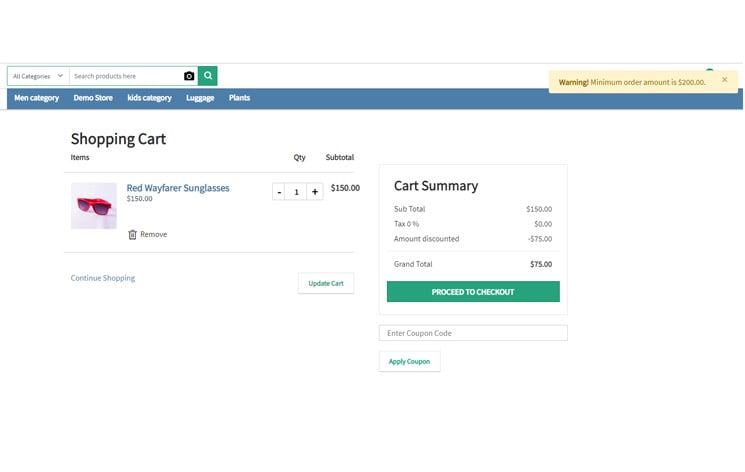On a clean white background, the upper left corner features a drop-down menu labeled 'All Categories' alongside a search bar for product searches. To the right of this, there's an image of a sleek black camera. Adjacent to the search bar, a conspicuous green square with a white magnifying glass icon invites users to search.

Towards the right-hand side, a pop-up window framed in yellow with a blue backdrop prominently displays the word "Morning" in bold orange text. Beneath it, a pertinent message in a white font states "Minimum order amount is $200," accompanied by a gray 'X' for closing the pop-up.

Below, a navigation bar in a blue background with white text lists categories: 'Men', 'Demo Store', 'Kids', 'Luggage', and 'Clients'. 

The central section presents a shopping cart overview on a white background with black text headings: 'Shopping Cart', 'Items', 'Quantity', and 'Subtotal'. Following this, an image of a stylish pair of red Wayfarer sunglasses is displayed. Next to the image, in blue text, reads the item name 'Red Wayfarer Sunglasses - $150', with a quantity field showing '1' and an individual price of '$150'.

On the right, a detailed cart summary in black text includes:
- 'Subtotal: $150' in gray
- 'Tax: $0'
- 'Amount Discounted: $9.75'
- 'Grand Total: $75'

Beneath the summary, options in blue text are available for 'Continue Shopping' or 'Update the Cart'. A green button at the bottom, with white text, prompts users to 'Proceed to Checkout'. Additionally, there is a box to enter a promotional code, with a corresponding button to apply it.

This image depicts a shopper encountering a message indicating a minimum order requirement of $200, thereby unable to proceed to checkout due to insufficient spending.